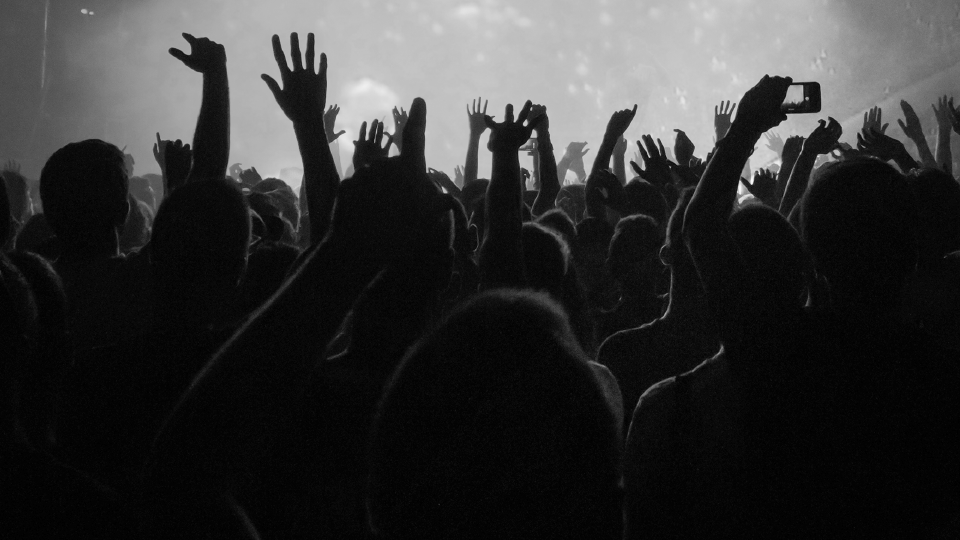The image is a striking black-and-white photograph capturing the energy and atmosphere of a live concert from behind the crowd. Shrouded in darkness and haze, the silhouettes of people's heads and hands form bold shapes against the overlit stage, emphasizing the enthusiastic participation of the audience. Variations in hand gestures—from all five fingers spread wide to fingers pointed toward the sky—create an engaging tapestry of movement. On the right, someone holds up a phone, its screen aglow, likely filming the performance. The intense, overexposed stage lights at the front obscure details of the performers, casting an ethereal glow and highlighting the edges of the crowd's bodies. The overall composition, including the smoky air and diverse silhouettes, conveys a powerful sense of unity and excitement among concertgoers, all intently focused on the vibrant energy emanating from the stage.